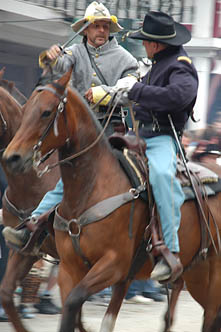This photograph captures two men riding brown, chestnut-colored horses, seemingly part of a parade or historical reenactment, likely of the Civil War era. The man on the left is dressed in a long-sleeve black shirt, blue jeans, and a black cowboy hat adorned with a gold string around its band. He is holding only the reins of his horse. The man on the right is garbed in a long-sleeve gray coat with a white hat that features an emblem of two crossed swords and an ax on the front. He is holding what appears to be a sword in his right hand. The background suggests a cityscape, and the bottom of the image reveals the feet of some spectators, adding to the impression of a public event. The detailed attire and props indicate a possible Civil War reenactment, with the men representing opposing sides, the Confederates and the Union.